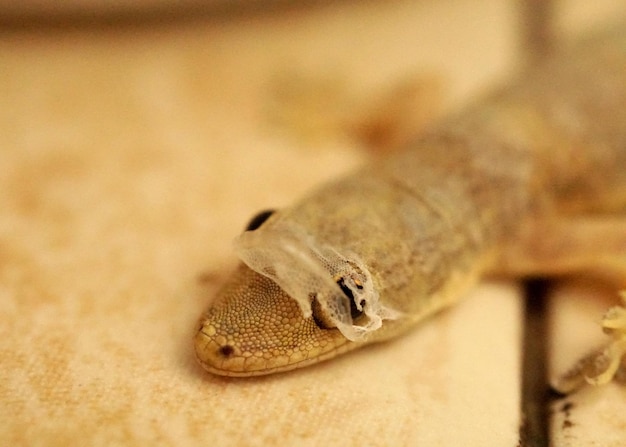The photograph captures a close-up of a brown lizard's head, which is in the process of shedding its skin. The primary focus is on the lizard's head and eyes, which are partially veiled by the peeling skin. The lizard's eyes are black and almost obscured by the shedding layer. The background is a blurred, uniform beige color, possibly a carpet or some neutral surface, making it difficult to discern what the reptile is resting on. The body of the lizard, extending from the upper right corner of the image, and its arms above and below the head are also blurred, preventing any detailed observation. The detailed markings of the lizard's scaly skin, including the spotted patterns on its snout, are clearly visible, highlighting the intricate texture of its shedding process.